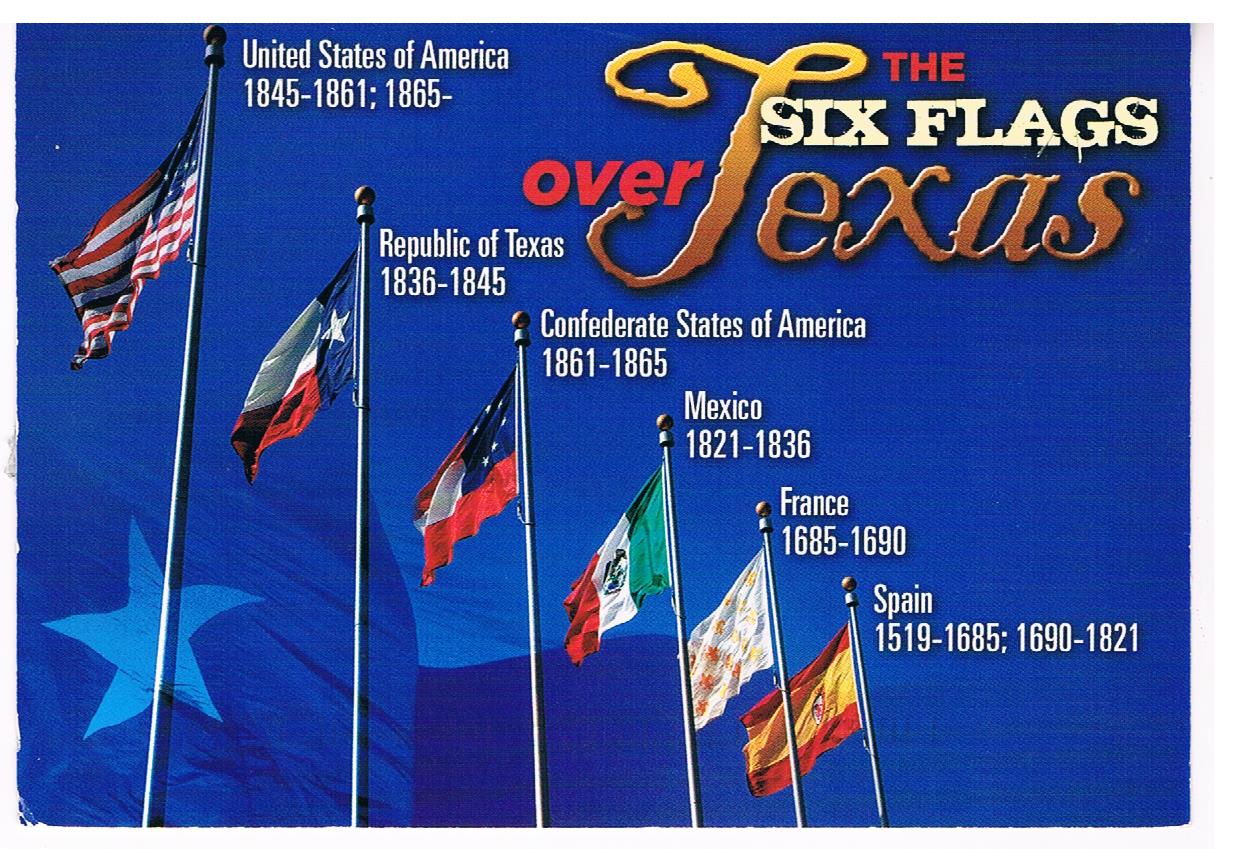The image is a vibrant close-up of several historically significant flags set against a blue background, accompanied by detailed text. Across the top of the image, in bold colors, it states "The Six Flags Over Texas." The title is spread out, with "the" in red text on the top right, "six flags" in white text just below, and "over Texas" split between red and yellow-orange text on the left side.

To the left, there is a sequence of flag images along with their corresponding historical details. The first flag is the United States flag, labeled in white text as "United States of America, 1845-1861; 1865-". Adjacent to it is the Republic of Texas flag, marked "Republic of Texas, 1836-1845." Following that, there is the Confederate States of America flag, with the dates "1861-1865." Next is the flag of Mexico, showing the period "1821-1836." The sequence continues with the flag of France, covering "1685-1690," and then Spain, denoted with "1519-1685; 1690-1821."

The various flags display a mixture of red, yellow, white, blue, and green, their vivid colors distinct against the blue backdrop. Though positioned in a static photo, the flags appear lively and dynamic, as if fluttering in the wind, evoking a sense of historical grandeur.